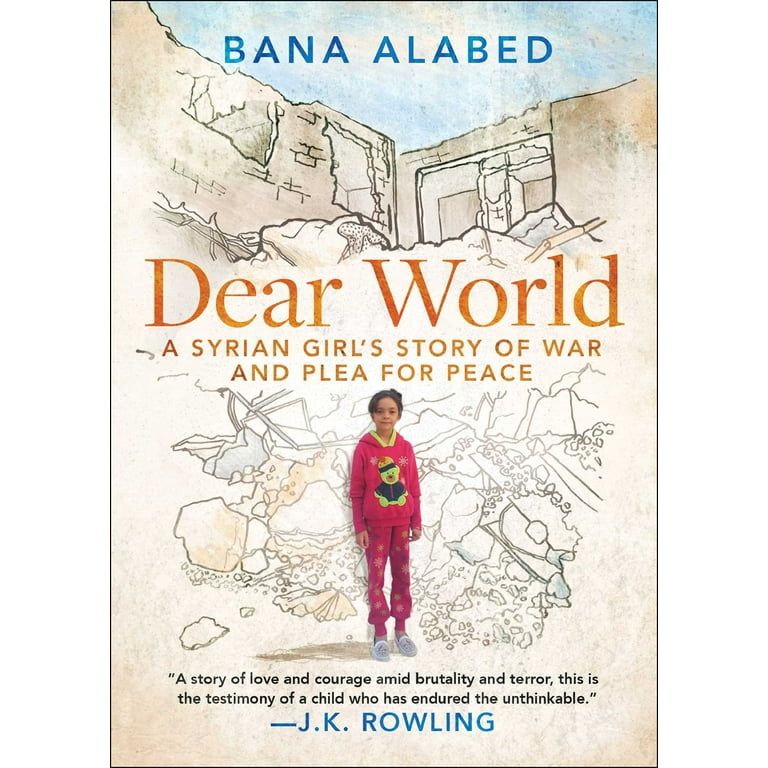The cover of the book features a detailed artistic drawing depicting a war-torn scene with a destroyed building, its remnants forming a large pile of rubble. The sky above is blue, contrasting with the destruction below. At the top, in blue letters, it reads "Bana Al Abed". Below that, prominently in the center, the title "Dear World" stands out in large letters, followed by the subtitle, "A Syrian Girl's Story of War and a Plea for Peace". Further down, a young girl dressed in red pajamas with a yellow bear imprint is seen standing amid the debris, highlighting her resilience and innocence. Above her, the book describes it as "A story of love and courage amid brutality and terror. This is the testimony of a child who has endured the unthinkable." At the very bottom, a note in red and blue letters credits JK Rowling for the foreword. The scene graphically underscores the stark reality of war, portraying both destruction and an indomitable spirit.